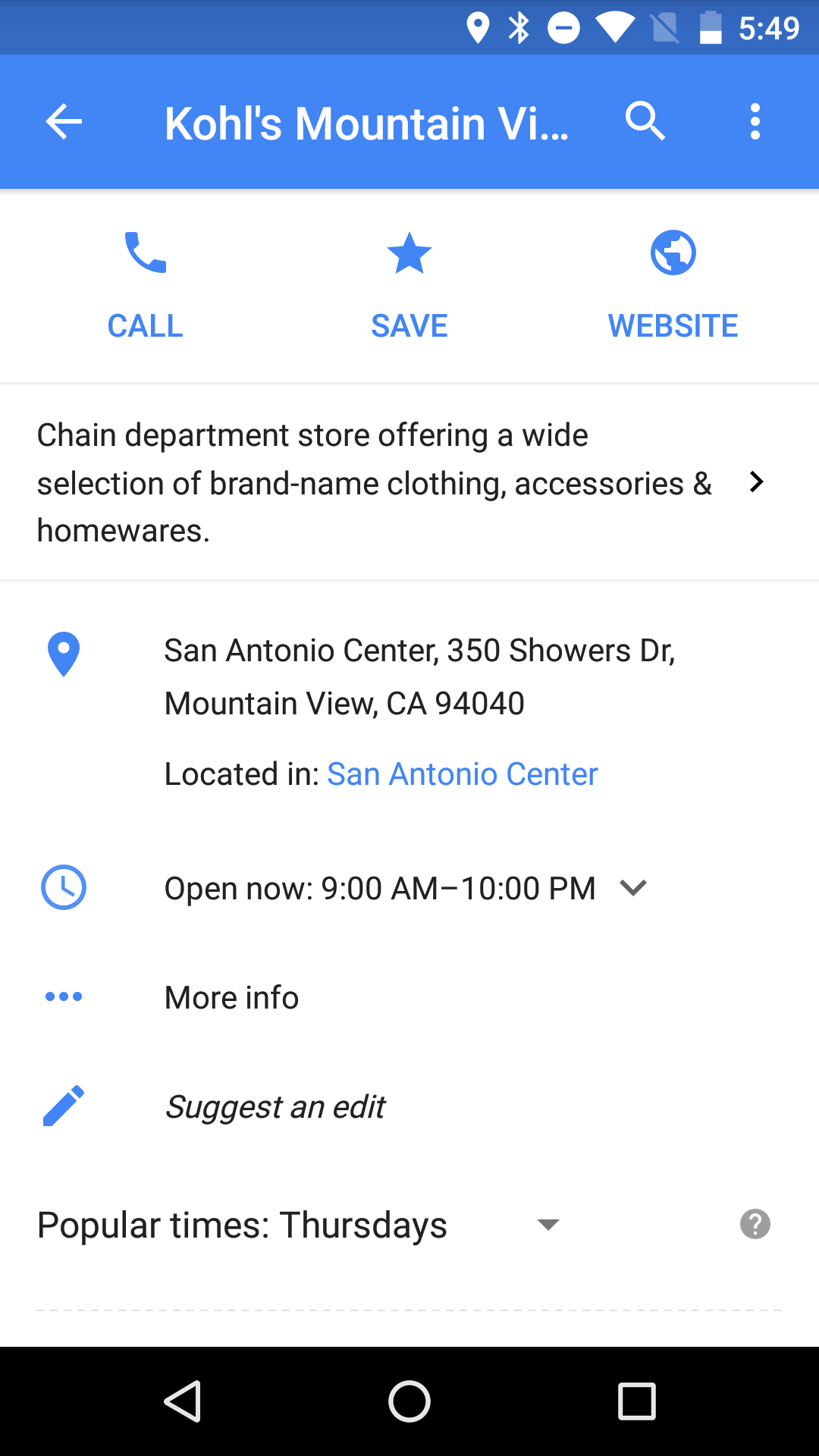The image features a structured layout on a white background. At the top, there's a darker blue box displaying the price "$5.49." Below it, a lighter blue box contains a left arrow, the text "Kohl's Mountain View," a magnifying glass icon, and three dots.

Further down, another white background section highlights the headings "Kohl's Save" and "Website," separated by a thin line. Beneath this line, a brief description reads: "Chain department store offering a wide selection of brand name clothing, accessories, and homewares," which is followed by a right arrow.

Continuing downward, there's another dividing line, below which a blue pin with a white center is featured. The text next to the pin reads "San Antonio Center, 350 Showers Drive, Mountain View, California 94040, located in San Antonio Center," highlighted in blue.

Adjacent to this, a blue clock icon indicates "Open now, 9am-10pm," accompanied by a down arrow. There are also three small blue dots labelled "More info," alongside a blue pencil icon with the wording "Suggest an edit." The section then notes "Popular times, Thursdays," with an additional down arrow.

On the right side of the image, a gray circle contains a question mark icon. Below it, a black box features a trio of icons: a triangle, a circle, and a square.